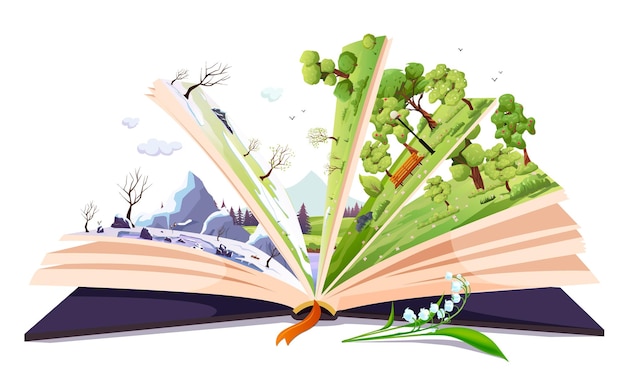This digitally illustrated image, presented in landscape orientation, resembles a pop-up book laid flat on a white surface. The cover of the book is deep purple, accented with a peach-colored ribbon bookmark emerging from the binder. The pages are light pink in hue and layered at various angles, revealing distinct seasonal scenes in the spaces between them.

On the far left, the first scene depicts a cold, wintry landscape with bare trees and snow-covered ground, reflecting a stark winter ambiance. The scene transitions to early spring in the central partition, where barren trees stand amidst patches of snow and emerging green grass. Moving rightward, the landscape becomes more lush and vibrant with trees gaining leaves and a noticeable increase in foliage. One of the rightmost partitions features a serene park scene complete with a bench, surrounded by fully green trees, symbolizing the height of spring. This seasonal progression culminates in a final scene filled with verdant trees, against a backdrop of distant mountains, clouds, birds, and a tranquil lake. Additionally, a small green stem bearing white flowers rests on the surface outside the book, as if it had just fallen out from one of its pages.